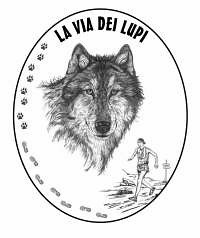This detailed illustration features an oval shape with a thin black outline. The image is rendered in black, white, and shades of gray. Centered within the oval is a striking depiction of a wolf, symbolic and detailed in its monochromatic palette. Above the wolf, the text "La Via Dei Lupi" is prominently displayed. This phrase translates to "The Way of the Wolves," hinting at the transformative journey depicted.

Starting from the bottom right corner of the oval, there is a figure of a person walking on what appears to be a dirt path. This figure's footsteps progress orderly along the left side of the oval. As these human footsteps continue upward, they gradually morph into canine paw prints, suggesting a metamorphosis from human to wolf. This transformation narrative is further emphasized by the paw prints leading up to the top left section of the oval, towards the text at the top.

Additionally, the illustration meticulously showcases various elements like the transitioning footprints and paw prints winding upwards to create a sense of movement and evolution within this artistic piece. The entire image captures a seamless blend of symbolism and artistry, portraying a poignant journey from humanity to the wild essence of the wolf.